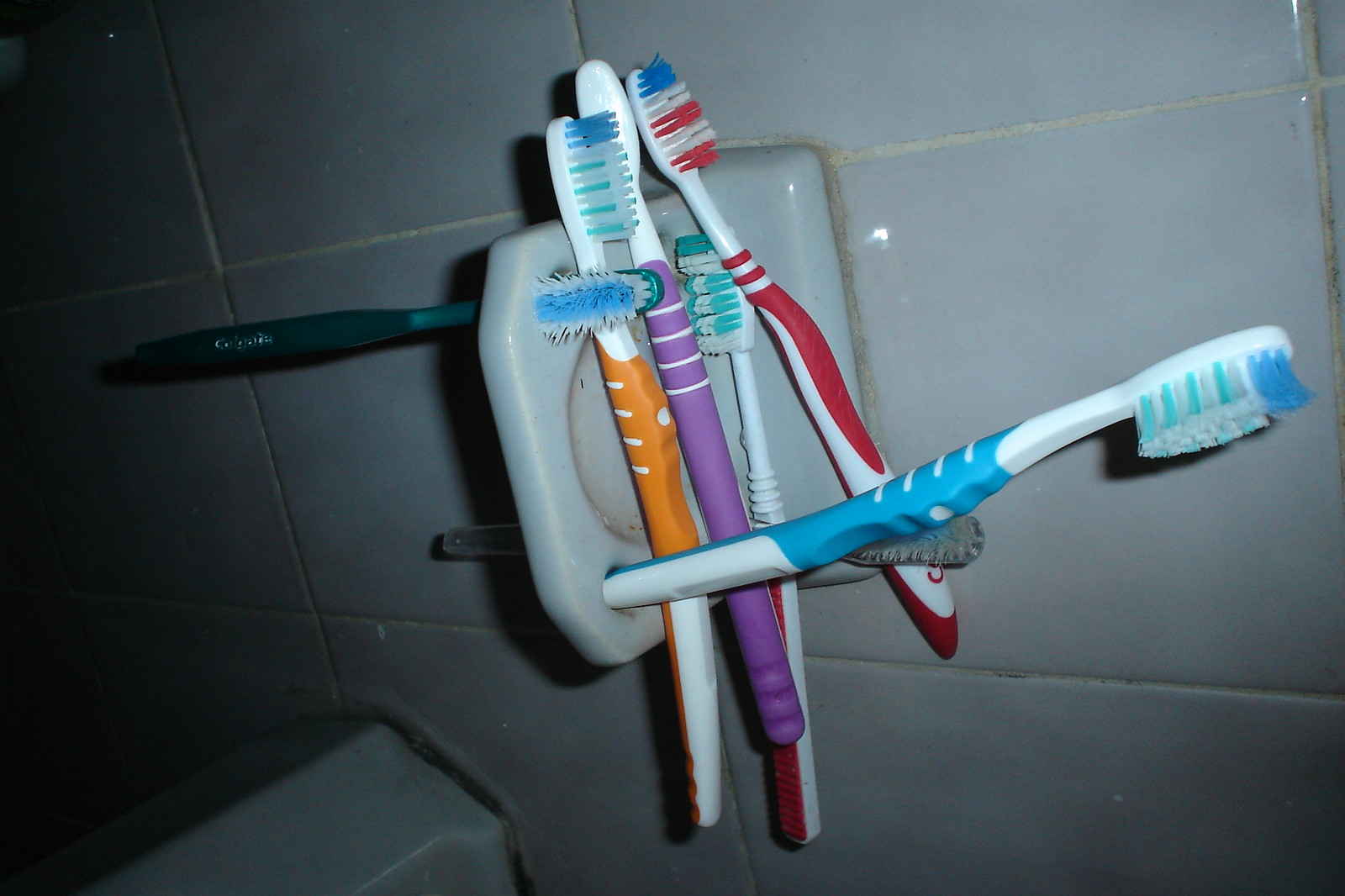This photograph captures a bathroom setting featuring a gray-tiled backsplash and a toothbrush holder attached to the wall. The toothbrush holder, also tiled in gray, is designed to hold toothbrushes upright but is angled to the side. It contains six toothbrushes in total. 

Four toothbrushes are haphazardly laid across the top, while two are inserted into the perforated holes, albeit one barely fits and sticks out. The toothbrushes display a variety of colors: two are red and white, one is blue and white, one is orange and white, one is solid green, and one is purple and white. The bristles of these toothbrushes are primarily white with variations that include teal, blue, and red highlights.

Two of the toothbrushes appear new and unused, while the bristles on at least three others seem significantly worn. In the background, white tiles adorn the walls, and shadows obscure parts of the left side of the image. A white object is also visible in the lower left corner, contributing to the overall bathroom theme.